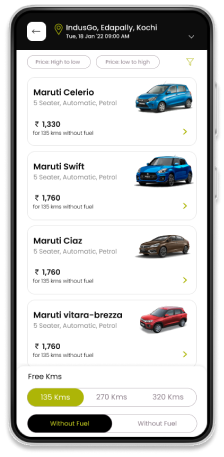This website page appears to be dedicated to car rentals or sales, featuring a selection of Maruti cars. It prominently displays the name "Lindisco Edapalli Kachi" with a challenging-to-read timestamp indicating both January 13th and January 18th, 2023, at 9 AM. The page is bordered by a black frame, and at the top, there are two indistinct ovals containing unclear information.

The main section showcases four Maruti car models, each placed within a white background and bordered by rectangles containing black text. The cars listed are:

1. **Maruti Celerio** priced at 1,330 rupees.
2. **Maruti Swift** priced at 1,760 rupees.
3. **Maruti Ciaz** priced at 1,760 rupees.
4. **Maruti Vitara Brezza** priced at 1,760 rupees.

The first two cars are colored blue, the third is a brownish gold, and the fourth car is red. Beside this list, there are distance options presented in bright ovals: 135 kilometers (highlighted in bright green), 270 kilometers, and 320 kilometers. Additionally, there is a selection at the bottom that states "without fuel," highlighted in black with green writing, suggesting that these may be options for electric or fuel-less rentals. The overall theme of the buttons on the page is primarily gray or white, with the exception of one green and one black button.